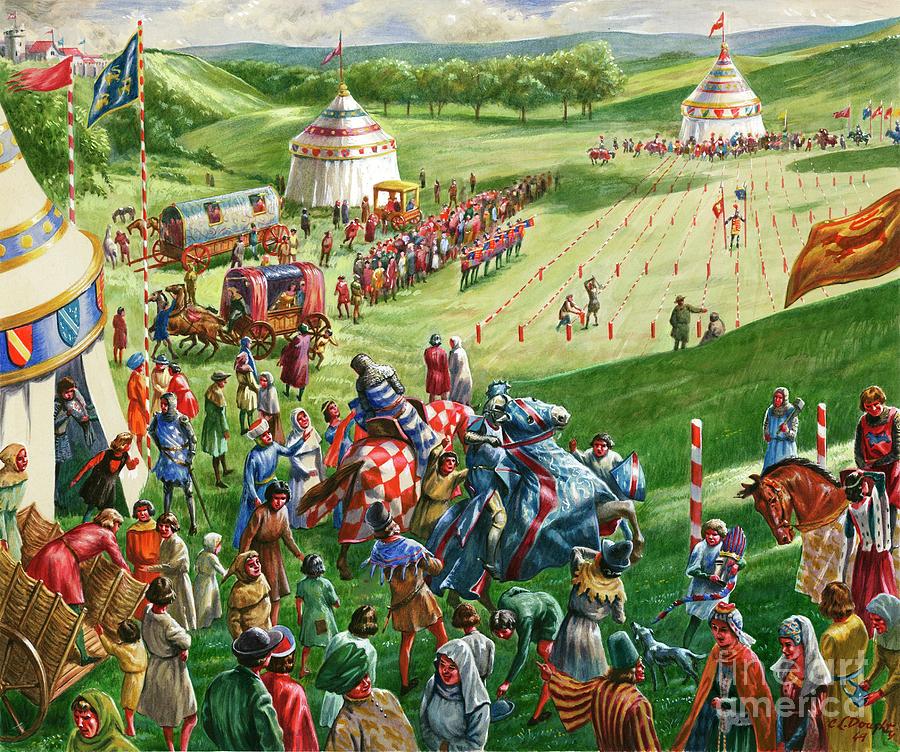This image is a detailed and colorful painting of a medieval tournament taking place in a vast, outdoor setting. The scene showcases large rolling green hills with lines of vibrant green trees and distant, majestic mountains under a blue sky filled with fluffy white clouds. Scattered across the expansive field are several large, white, circular tents adorned with brightly colored pointed tops in hues of red, blue, and green, each topped with a fluttering flag. 

In the background, towards the right side of the image, there is a central clearing marked by parallel lines of barriers set up for jousting. People are gathered around these barriers and seated to the left, watching the activities. In the foreground, a lively crowd is dressed in medieval attire—many in robe-like garments, while some are donned in armor and mounted on horseback, seemingly readying for a jousting contest.

Amidst the bustling crowd, a few caravans, one notably with holes cut for people to look out, are present, along with wagons, including one from which a woman is observing the scene. The sense of anticipation is palpable, as it appears the crowd is eagerly awaiting the start of a jousting display. The crowd's atmosphere, combined with the detailed depiction of medieval life and the vivid scenery, lends a lively, festive air to this historical reenactment.